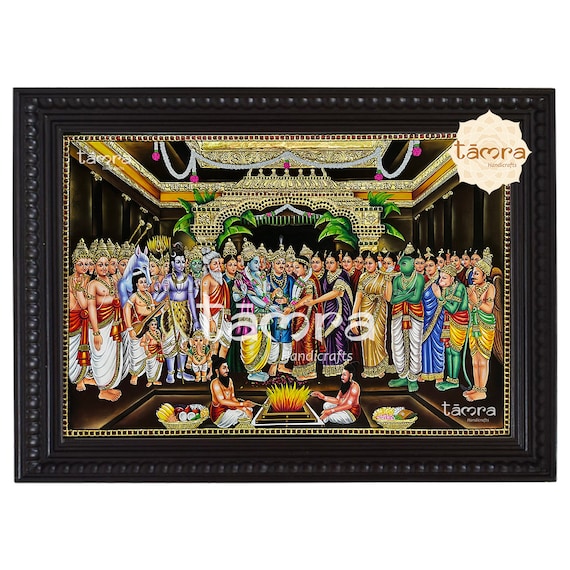The image showcases a bright, vibrant painting framed in a textured black frame with a gold inner edge. The artwork depicts an elaborate scene resembling a religious or celebratory gathering. The background features an ornate archway or gate, flanked by palm trees, suggesting the scene takes place in a grand, dark room. In the foreground, two bearded men with their hair tied up are seated around a fire pit, appearing engaged in roasting food. Behind them, numerous baskets overflow with various fruits and foods. Surrounding the fire pit, a multitude of figures, possibly up to 50 or 60, dressed in Roman-style robes and extravagant gold headdresses, many of which are god-like figures with blue or green hues, indicating a possible portrayal of Indian deities such as Krishna. The scene is rich with color and detail, emphasizing a festive or sacred atmosphere. Notably, there is a stamp labeled “Tamra” in both the upper right and lower right corners.